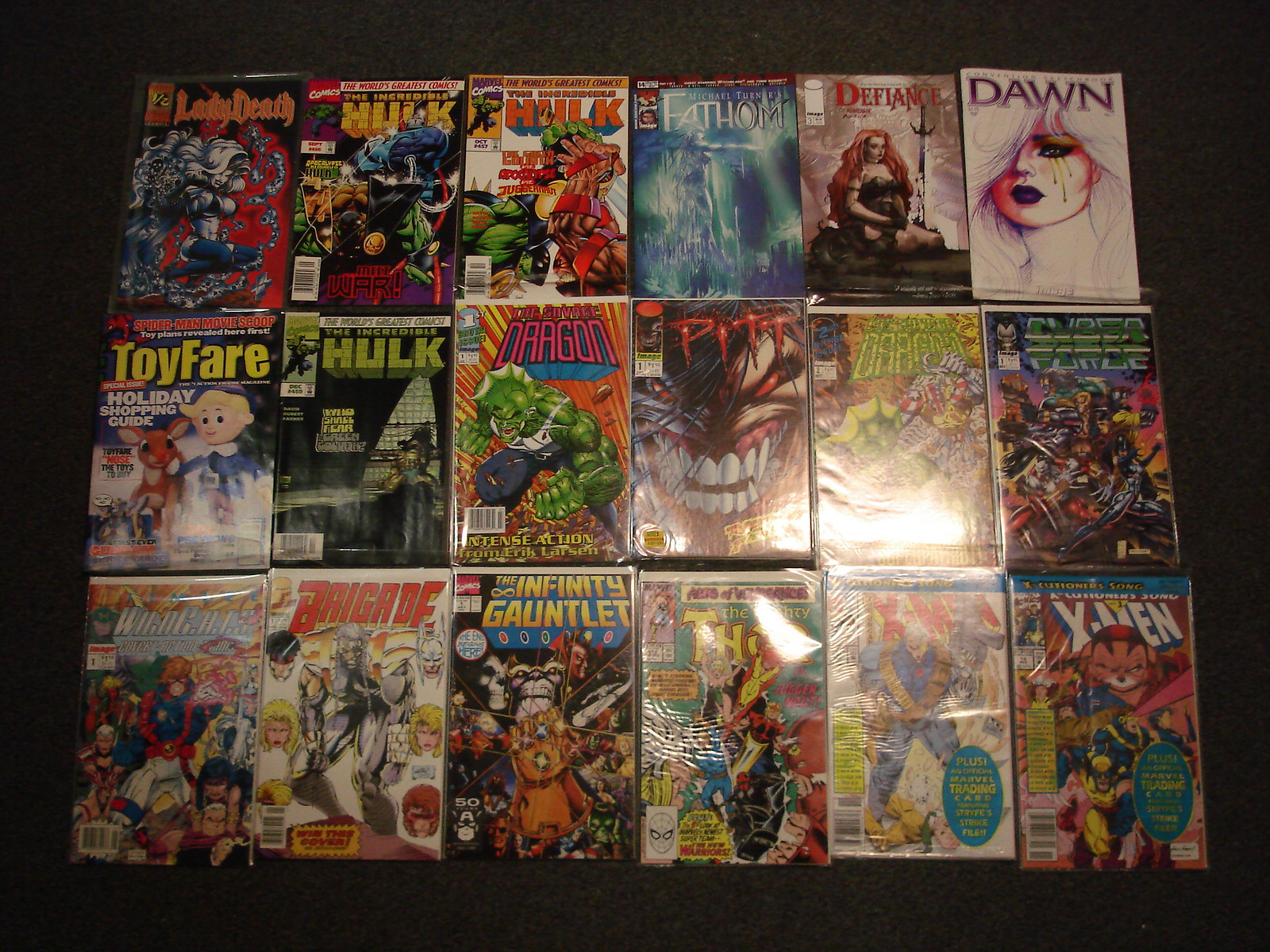This image depicts a meticulously arranged collection of 18 comic books, neatly laid out in a grid with six comics per row, across three rows. Each comic book boasts a brightly colored, vividly detailed cover featuring a variety of iconic characters. Starting from the left in the first row, the comics include titles such as Lady Death, The Hulk, Fathom, Defiance, Dawn, and Toy Fair Hulk. The second row features comics like Dragon, Pit, another depicting a dragon, Wildcats, and Brigade. The final row showcases additional titles, including another Hulk, X-Men, Spider-Man, and an indeterminate comic possibly named Infantry Gauntlet. Each comic cover presents unique, eye-catching artwork representative of its story and characters.